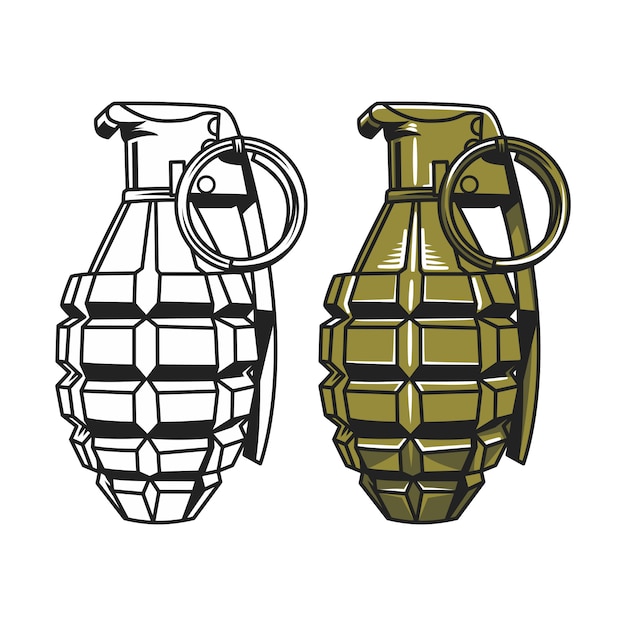This digital illustration, reminiscent of clipart style, features two identical drawings of a hand grenade placed side by side against a white background. The left image is a black-and-white outline, showcasing detailed shading at the bottom, near the center grips, and beneath the pin mechanism. The right image mirrors the left but is colored in a dark olive green. The same black shading is preserved, while additional white highlights accent the pin and the sides. The grenade's texture and key features, such as the ring and pin, are clearly depicted in both versions, with the right side adding more visual depth through selective coloring without filling in the pin, giving natural highlights throughout the illustration.